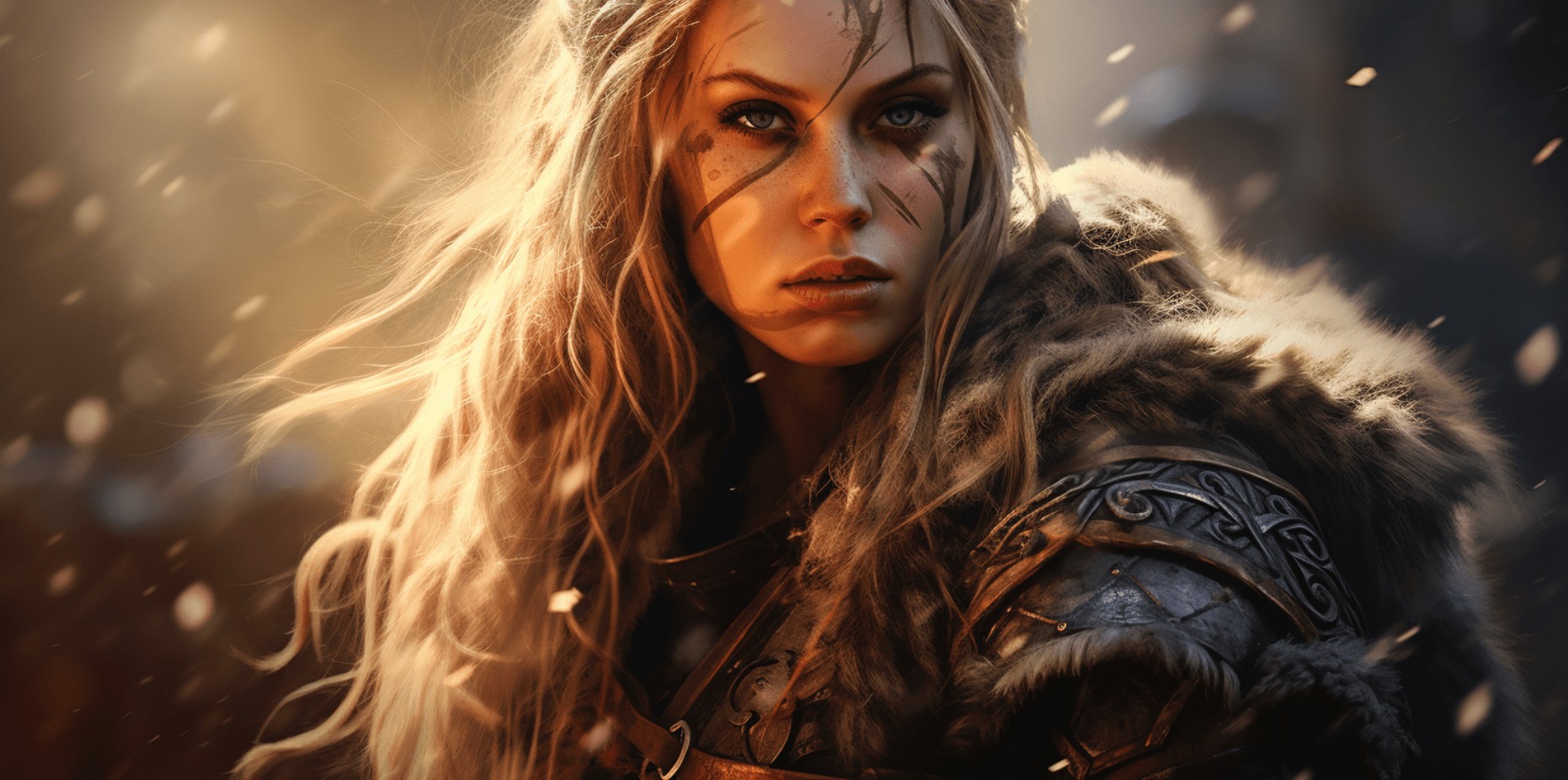The image depicts a stern-faced, warrior-like elf woman as the central focus. With long, wavy blonde hair cascading over her shoulders, she gazes intently ahead. Her white complexion is adorned with streaks of mud or paint, which add to her fierce demeanor. The woman is clad in a combination of leather armor and a fur-trimmed hooded cape, with visible metal shoulder pads contributing to her rugged appearance. The background of the image is an artistic blur of dark and light hues, filled with glowing specks reminiscent of sparks or embers from a fire. The overall atmosphere suggests an intense, possibly post-battle scene, enhanced by the contrast of bright light illuminating her from one side and shadow enveloping the other. Her piercing blue eyes further emphasize her resolute and unyielding expression.